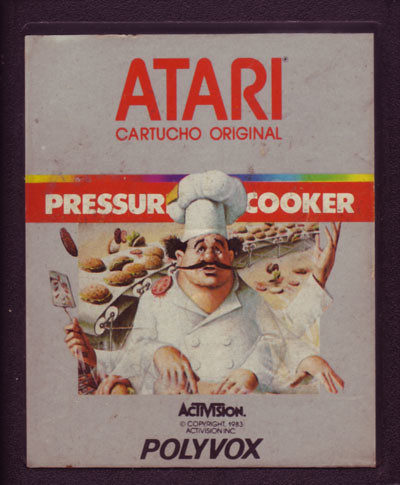This image features a vintage Atari game cartridge case set against a dark background. Dominating the top of the case is the iconic Atari logo in bold, red letters, with "Cartusia Original" inscribed just below it. Central to the design is the game title "PRESSURE COOKER" prominently displayed in all caps, in white text against a vibrant red ribbon. Below the title, a colorful cover art depicts a cartoon chef with a long, thin mustache and tufts of black hair peeking out from beneath a tall, white chef's hat. The chef's anxious expression is directed towards the viewer. Remarkably, he has multiple hands, each engaged in different culinary tasks - one holding a spatula, another seemingly handling bread, and possibly a knife in a third hand. The dynamic scene includes a conveyor belt with various plates of food, adding to the chaos. Surrounding the cover art is a black border, and beneath it are the logos for Activision and Pollywogs, along with the text "© 1983 Activision, Inc."